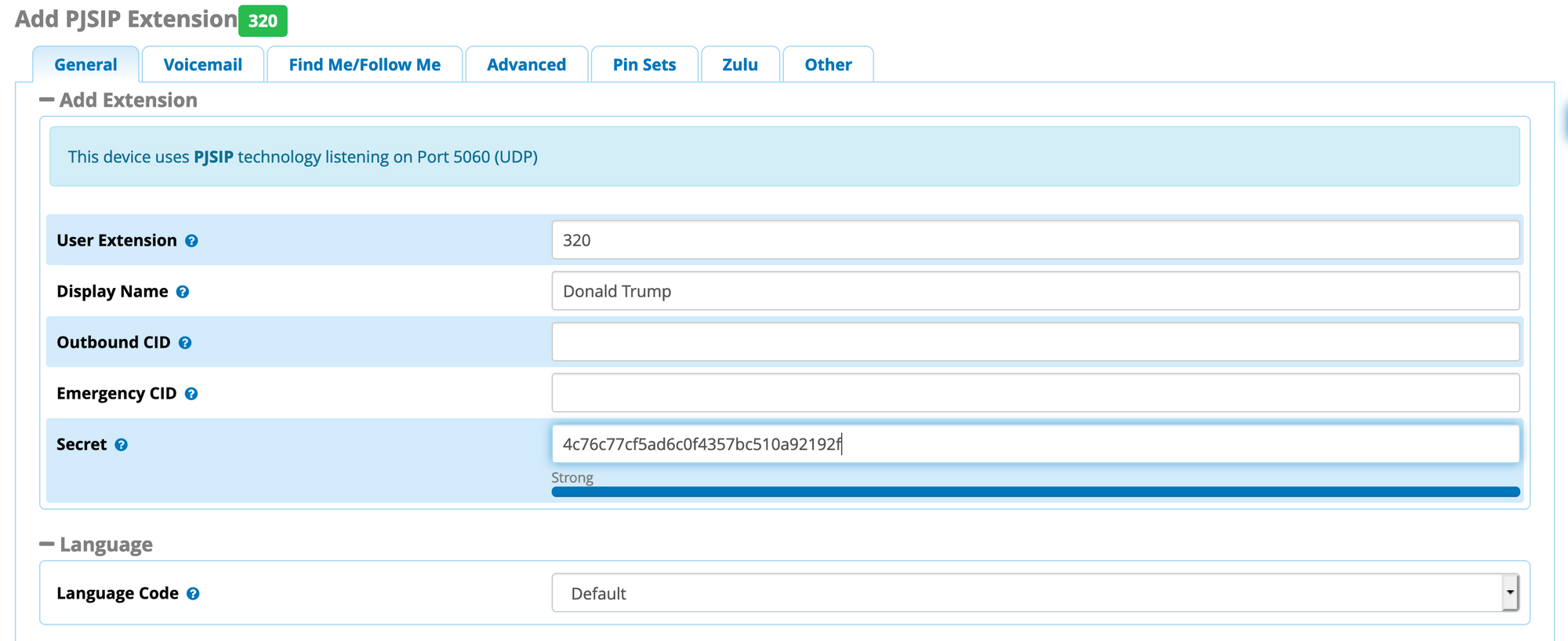In this image set against a white background, we see a horizontally extended screenshot. In the upper left corner, there is bold gray text that reads "Add PJSIP Extension," accompanied by a small green box labeled "320." Beneath this heading, a series of tabs are laid out horizontally, from left to right: "General" (which is the currently open tab), "Voicemail," "Follow Me," "Find Me," "Advanced," "PIN Sets," "Zulu," and "Other."

Within the open "General" tab, gray text indicates "Add Extension" at the top. Just below, a blue banner states, "This device uses PJSIP technology listening on port 5060 UDP." Vertically aligned beneath this banner are fields labeled "User Extension," "Display Name," "Outbound CID," and "Emergency CID." The interface appears to be part of a configuration or management system for telephony or VoIP services, specifically using PJSIP technology.